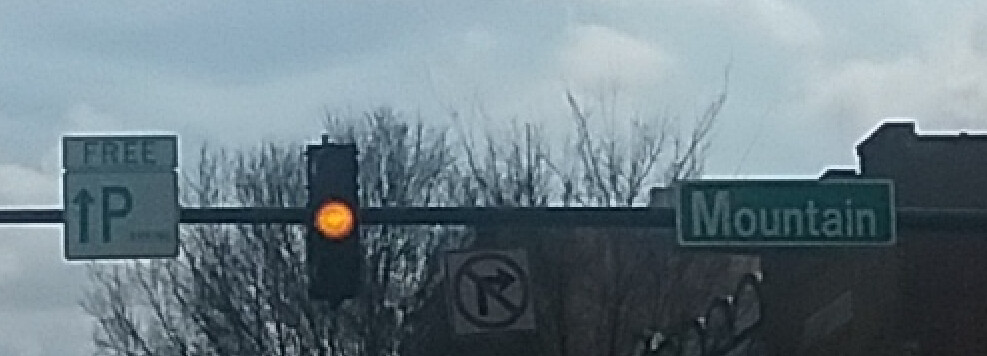The image depicts an outdoor scene on a street, framed from a low angle looking up. Dominating the scene is a horizontal street pole running from right to left. Attached to the pole in the center is a rectangular traffic light currently showing yellow. On the left side of the pole is a white square sign with the word "FREE" at the top, an upward-pointing arrow, and a large black capital "P," indicating free parking. On the right side, a green street sign with a white border reads "Mountain," with the "M" capitalized.

In the background, the tops of some leafless trees are visible, suggesting the scene might be set in late autumn or winter. Behind these trees, there is a large, brownish building on the right side of the image. The sky above is a mix of blue-gray with some white-gray clouds scattered throughout. Near the bottom center of the image, there is a white square sign featuring a red circle with a diagonal slash over a black arrow curving to the right, indicating no right turn. The overall atmosphere is one of a cloudy, possibly cold, day.